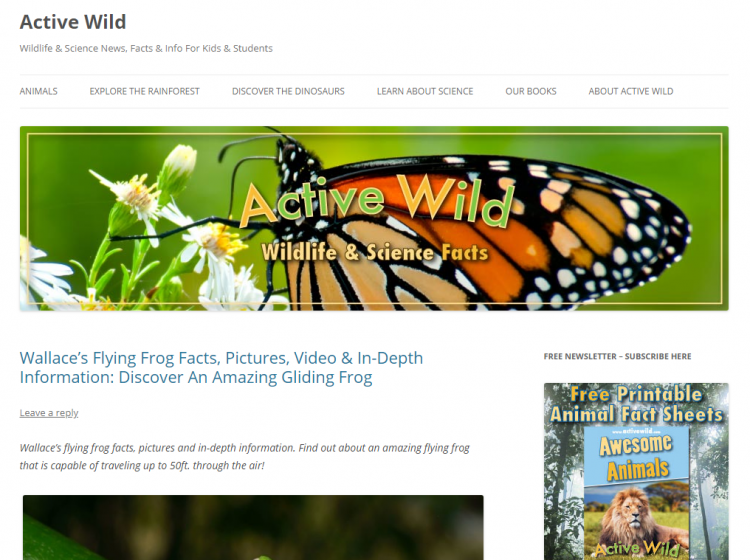The desktop homepage of the Active Wild website, renowned for its wildlife and science news, facts, and information specifically tailored for kids and students, showcases vibrant and engaging content. The main sections of the website include categories like "Animals," "Explore the Rainforest," "Discover the Dinosaurs," and "Learn About Science," as well as a collection of books published by Active Wild.

Dominating the homepage is a striking, wide-angle image of a butterfly perched on a flower. The butterfly, an adult with black and orange wings, is shown in exquisite detail. 

Beneath this image, a section titled "Wallace’s Flying Frog Facts" promises fascinating insights, pictures, videos, and comprehensive information about an extraordinary frog species known for its gliding abilities. A teaser snippet informs readers that Wallace's flying frog can glide up to 50 feet through the air.

The overall background of the website is white, with most of the text in black, ensuring a clean and easy-to-read presentation. To the right of the page, there are two prominent calls to action: a "Free Newsletter" subscription sign-up, and a link to "Free Printable Animal Fact Sheets," featuring an alluring image of a lion lounging in the savanna. This content, clearly aimed at a younger audience, highlights some of the more captivating and popular animals that are likely to appeal to kids' interests.